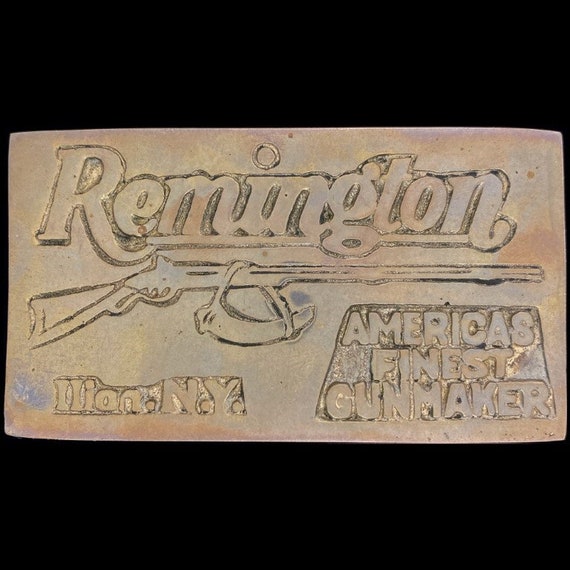The image shows a worn, patinaed metal sign for Remington, likely made of iron, and boasting a rusty, silver-copper sheen. Set against a black background, the sign prominently displays the text "Remington" at the top, with "Illion, New York" in the left corner and "America's Finest Gun Maker" in the right corner, all etched into the metal. The center of the sign features a detailed engraving of a Remington rifle with a powder horn hanging from the barrel, suggesting its antique nature. Despite visible grime, corrosion, and scuff marks, the sign retains a certain grimy charm, reflecting its historical significance and weathered beauty.